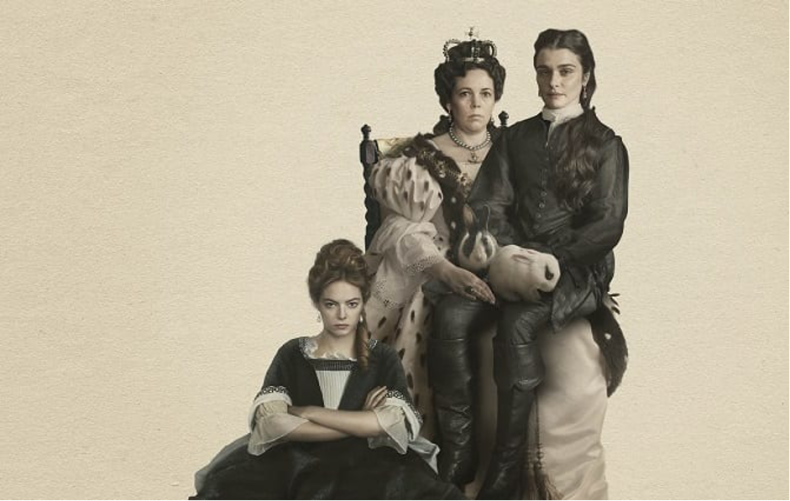This black-and-white image, reminiscent of the early 1800s, depicts three women in historical attire, posed in a rectangular frame that is wider than it is tall. At the center, an older woman, likely a queen, sits on a high-backed throne-like chair. She wears a crown and a white dress with polka dots, adorned with lace at the elbows, and a striking necklace. Her expression is one of displeasure.

Sitting on the queen's lap is a young woman dressed in dark clothing, possibly pants and boots, who holds two rabbits. This woman, with black hair, appears more content than the others. To the front-left of the queen, a teenage or young adult girl sits on the floor with her arms crossed, dressed in a green velvet dress with lace accents and a white design. Her expression is one of clear anger or frustration. The background is a simple cream color, adding to the vintage and formal atmosphere of the portrait.